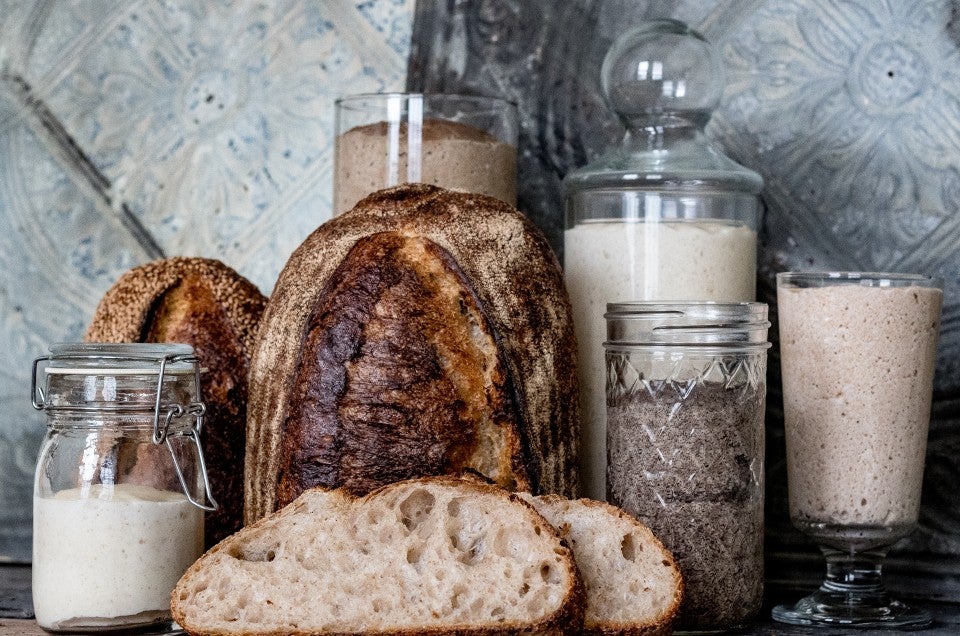The image showcases an assortment of artisanal bread and various food mixtures elegantly arranged on a table against a blue, floral-patterned wall. At the center stands a loaf of freshly baked bread, its golden crust contrasting with the soft beige interior, from which two slices have been cut and placed in front. To the left of the main loaf, there's a smaller oblong loaf adjacent to a wire-lock jar containing a white substance, possibly flour or milk. Directly behind the central loaf is a glass jar containing a brown mixture, likely a form of yeast or dough starter. To its right, another jar with a brown ball-shaped handle is filled with a white mixture. In front of this is a jar with diamond etching, harboring a dark brown substance, possibly a type of seasoning or molasses. On the far right, a clear glass holds a pinkish-brown mixture. The collection of transparent jars and glasses, each containing a different mixture or seasoning, along with the deliberately arranged loaves of bread, gives the scene a meticulously curated, magazine-worthy aesthetic.